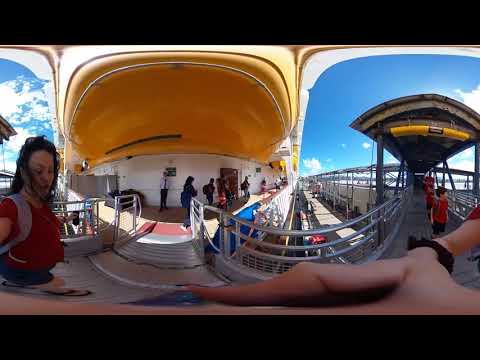In this image, numerous people are preparing to board a large cruise ship. The ship, sprawling in both directions, features a yellow ceiling or possibly an overhead yellow life raft. The scene is set on a metal overhang walkway above a wooden boardwalk. Several individuals are visible, with four or five people walking along the side of the ship and additional people in the foreground. One prominent figure in the foreground is a woman dressed in summer attire, wearing a red shirt, shorts, sandals, and a backpack. She appears to be looking downward. There's also a person holding a camera with their right hand, seemingly entering from the wooden walkway towards the ship. The photo captures a bright daytime setting with blue skies and minimal clouds.

The image employs a 360 framing technique, as evidenced by special effects that merge parts of the person on the left side into the right side of the photo, creating a seamless panoramic view. The person taking the selfie wears a black watch, which is visible at the bottom of the photo. The top and bottom of the image are bordered by black rectangles, adding a cinematic feel to the scene. The railings alongside the walkway are designed to prevent people from falling into the water, reinforcing the impression that the photo captures the moment just before boarding the ship.